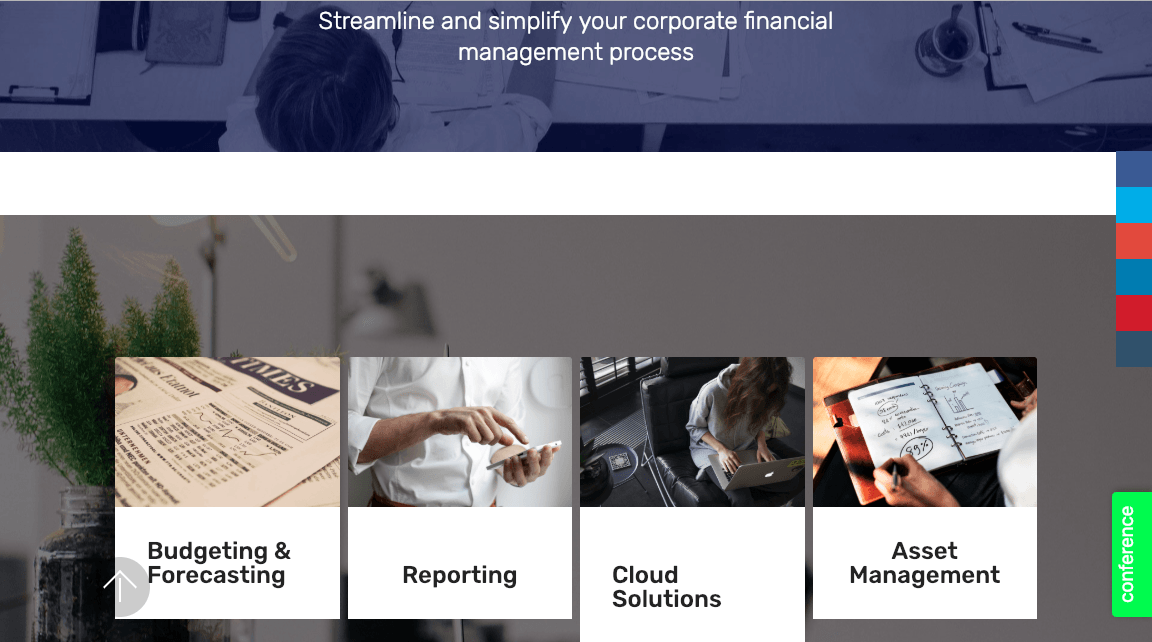This screenshot is from the top section of a business website's page. The background features a gradient from light to dark blue. The main image shows a man sitting at a desk. To his right, there is a coffee cup, a pen, and a notepad. On his left, notepads are arranged. The prominent white text reads: "Streamline and simplify your corporate financial management process."

Below this section, the background switches to white, followed by a gray area displaying additional elements. On the left, there is a small plant and a lamp behind it. This section highlights four service options: Budgeting and Forecasting, Reporting, Cloud Solutions, and Asset Management, each within its own box accompanied by supportive images. 

- Budgeting and Forecasting is represented by a newspaper image.
- Reporting features an image of a man pointing at a phone.
- Cloud Solutions shows a woman sitting at a desk.
- Asset Management has an image of a person writing in a daily planner.

To the right of these descriptions, there are square, color-coded boxes forming a decorative border. The colors alternate in the sequence: dark blue, light blue, light red, blue, blue, red, and dark blue.

Near the bottom, there is a small green tab with white text that reads "Conference."